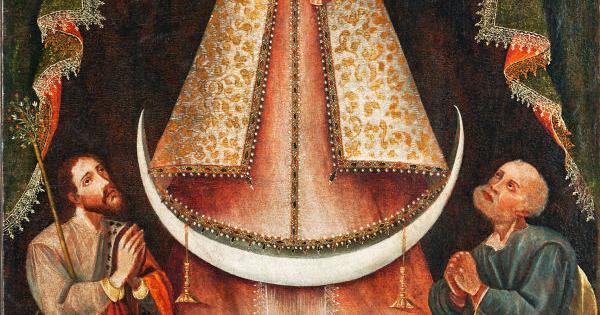The image depicts a detailed and ornate scene likely originating from an antique painting or religious artwork, possibly showcased in a museum. The background is a deep black adorned with rich, green curtains, accentuated with white lace and beaded fringes. At the center of the composition, a large, triangular shape looms, suggesting the lower portion of a robed figure, likely representing Mary with her child. This figure's robe is opulent, featuring golden embroidery and a yellow paisley design against a white background with black edging and a red base interwoven with gold.

Flanking this central figure are two men, each in prayerful reverence. To the left, a man with short brown hair, a brown mustache, and a goatee wears brown attire and clutches a stick adorned with multicolored gems. A candelabra with a single candle is situated beside him. On the opposite side, a man dressed in a green robe with red trim and a white shirt also holds a prayerful pose. Both men gaze upward towards the robed figure, encapsulating the scene's sacred and reverent ambiance.